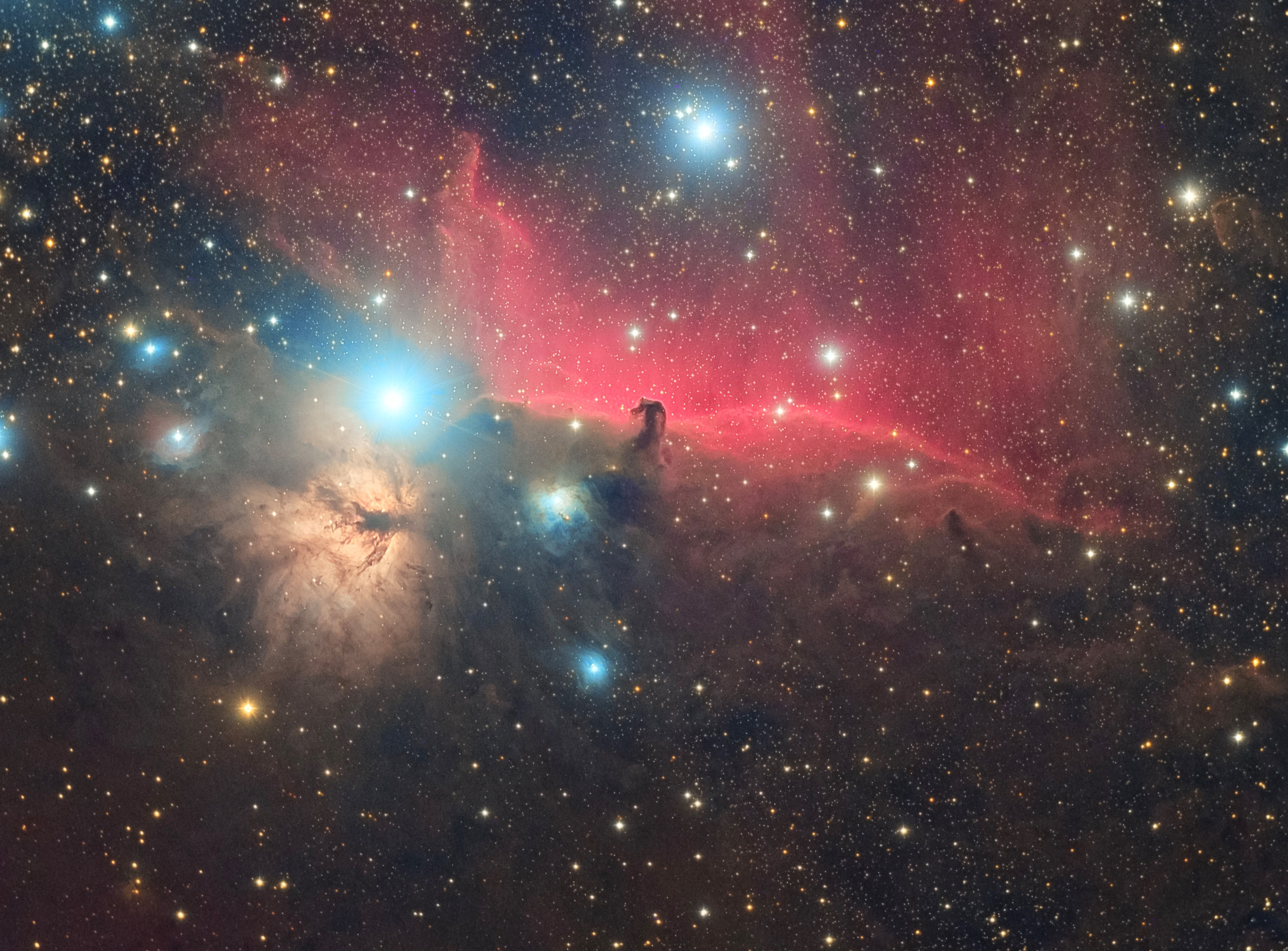This detailed photograph depicts the iconic Horsehead Nebula set against a backdrop of outer space, likely captured by the Hubble Space Telescope. Dominating the center of the image is the famous Horsehead Nebula, a striking red celestial structure with a distinctive horse head shape facing left. Surrounding this fascinating nebula are large, luminous stars, with some appearing vivid blue and others more muted yellow. The photograph also features countless tiny stars scattered throughout, creating a dazzling, star-filled expanse. Alongside the nebula, intricate gas clouds transition from pinkish and reddish hues at the top to darker, more organic tones below. The image is teeming with celestial details, including other smaller but less prominent nebula structures to the right, all contributing to the grandeur of this vast stellar landscape.